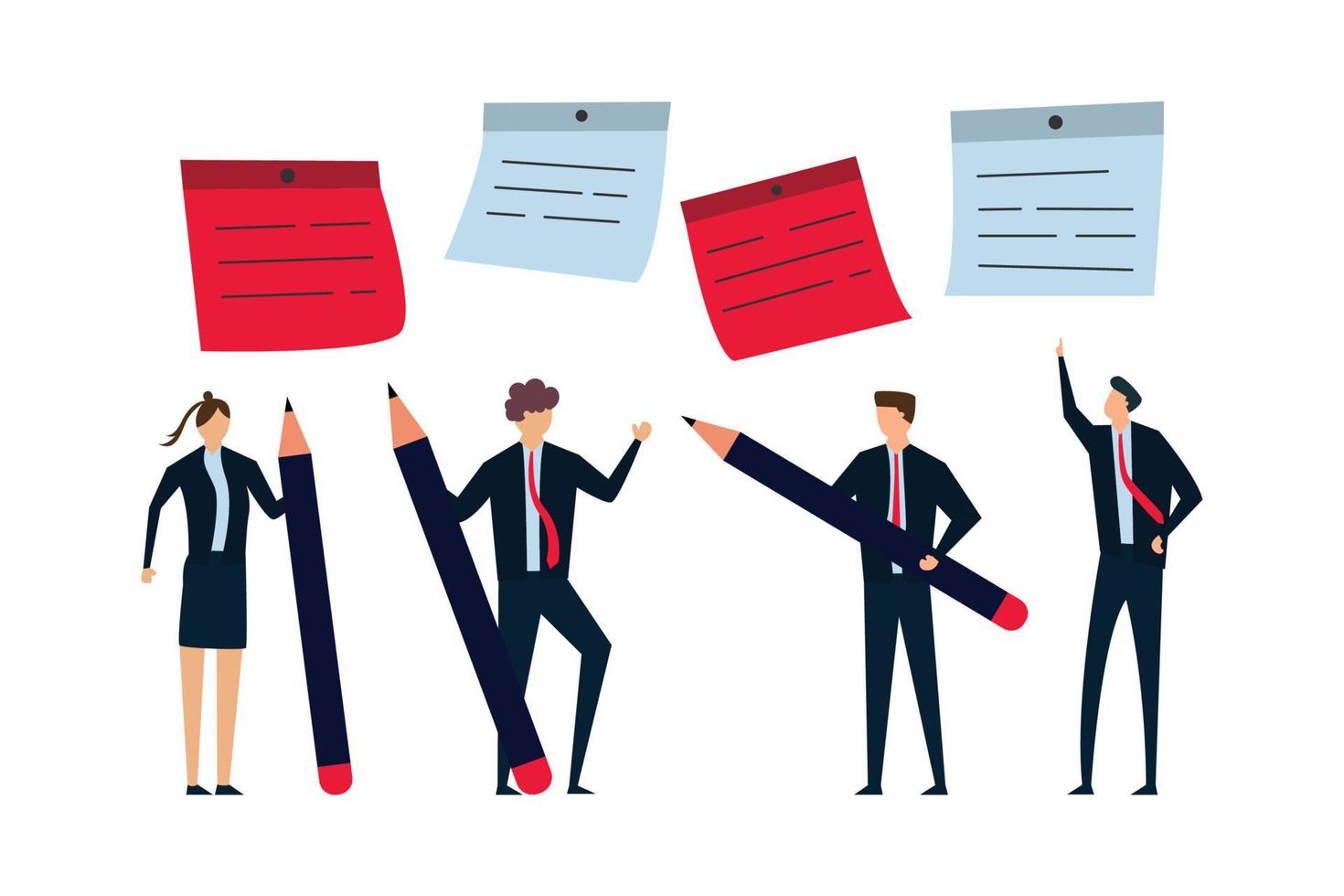The image is a detailed character sketch featuring four people against a plain white background with no visible borders. There are three men and one woman, all dressed in black or navy suits with light blue shirts. The men sport red ties. Each character holds a human-sized pencil, except for one man who is pointing upward. Starting from the left, the woman has brown hair styled in a ponytail and is dressed in a dark navy dress jacket and skirt over a light blue blouse. She holds her pencil in her left hand, pointing upwards. Next to her is a man with curly brown hair, also in a navy suit, light blue shirt, and red tie, holding his pencil in his right hand at a slight angle towards her. The third character, a man with short brown hair, is dressed similarly and holds his pencil with both hands, pointing it toward the man on his left. The final character, a man in an identical outfit, is looking upward and pointing at a red sticky note above his head. Above the characters, four sticky notes are displayed in a sequence: red, blue, red, and blue. These sticky notes have lines indicating writing, but no actual words are visible. None of the characters have detailed facial features, focusing instead on their outlined forms and colored attire.